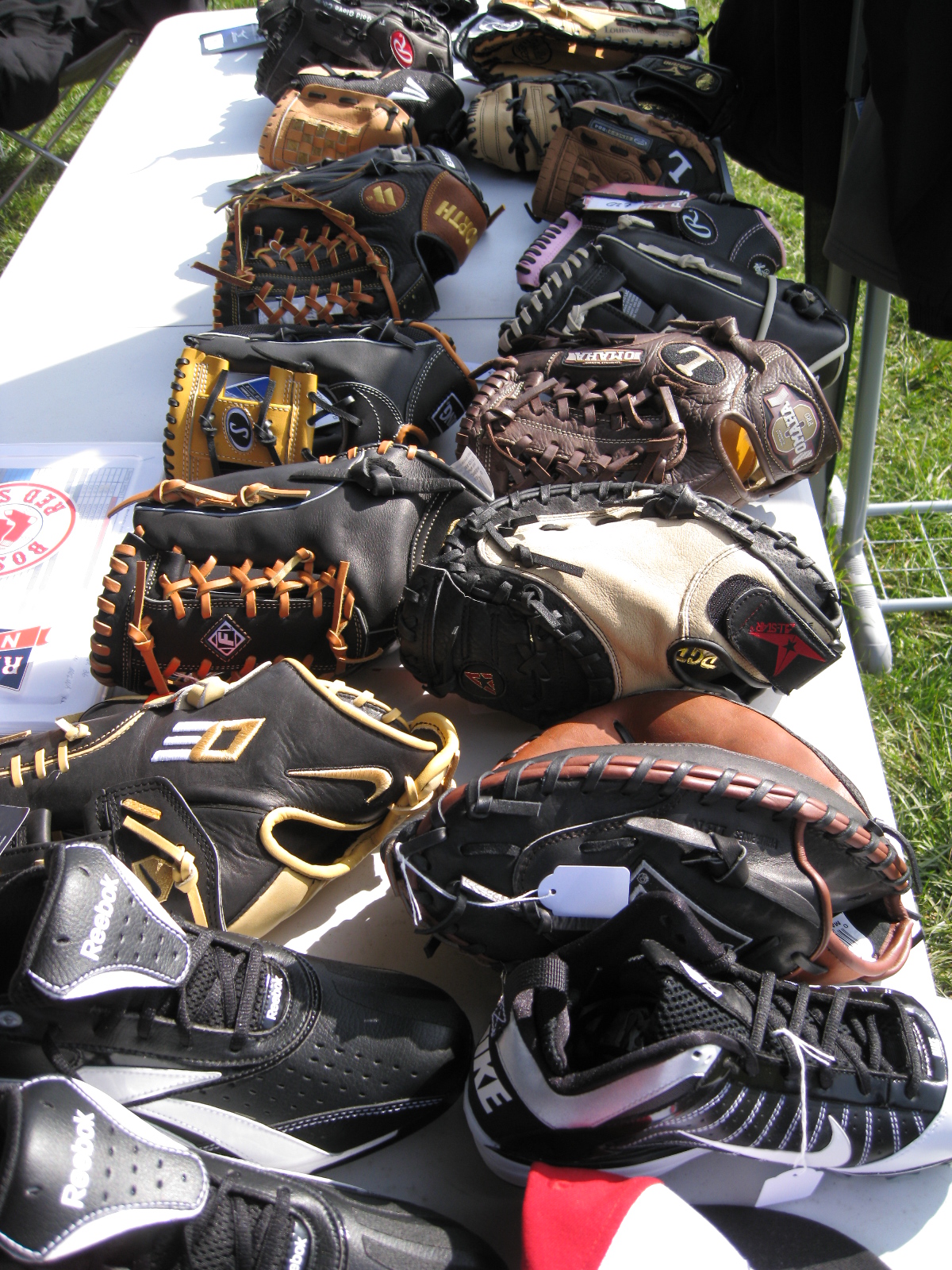An outdoor yard sale table sits on a grassy lawn, laden with various sports equipment. Dominating the foreground, a pair of black Reebok sneakers with white designs and black-and-white Nike tennis shoes catch the eye, each adorned with small sales tags. Towards the back of the white covered table, a collection of leather baseball mitts, including catcher's mitts and standard gloves of varying sizes, colors, and brands, are meticulously arranged. Some gloves bear the capital letter "L". To the left of the table, a piece of paper featuring the Red Sox logo is visible, while a black tag marks the top left corner of the setup. In the yard's background, just within sight, there is a rack hinting at more yard sale items.